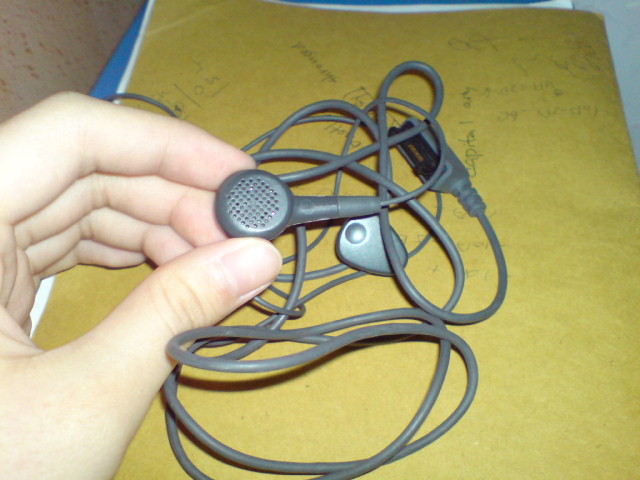The photograph captures a close-up of a person's left hand entering the frame from the left side, holding a single gray earbud. The visible fingers include the thumb and several other fingers, while the rest of the hand is out of the shot. The earbud has several small holes and a triangular piece, and it's connected to an old, tangled gray cord ending in a wide, retro-style adapter. The background features a yellow-colored folder with some indistinct green writing on it, possibly math work, though the text is too blurry to read clearly. Additionally, a blue folder appears to be underneath the yellow one, both resting on what seems to be a table surface. The primary focus of the image is the gray earbud held up against the folders, drawing attention to its detailed design and retro connector.